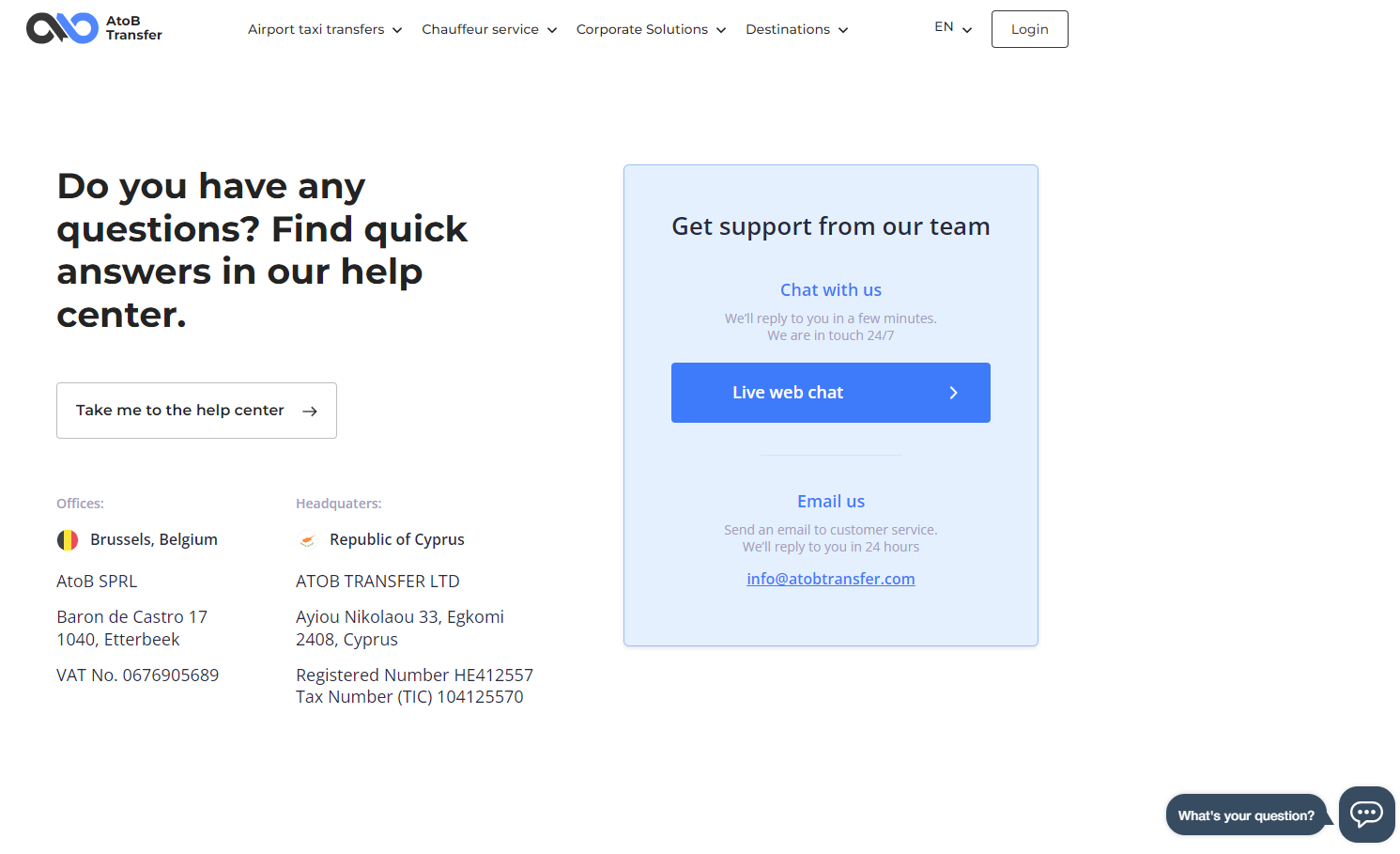The image showcases the ATOB Transfer website, prominently displaying its logo, which features an infinity symbol tilted on its side with a dual color scheme—blue on one side and black on the other. At the top of the webpage, there is a navigation menu offering options such as "Airport Taxi Transfer," "Chauffeur Services," "Corporate Solutions," and "Destinations." 

In addition, there is an "EN" language indicator next to a drop-down menu for language selection, as well as a "Log In" button. Below, a prompt invites users to find quick answers in the Help Center, accompanied by a button labeled "Take me to the Help Center."

The footer provides detailed contact information including offices located in Brussels, Belgium (ATOB SPRL, Baran de Castro 17, 1040 Etterbeck, VAT number 0676905689) and headquarters in the Republic of Cyprus (ATOB Transfer Ltd., AYIOU-NIKOLAOU 33, EGKOMI 2408, Cyprus, registered number HE412557, tax number TIC-104125570).

On the right side of the page, a support section offers users the option to get assistance from the team with a "Chat with us" feature, highlighted by a blue button labeled "Chat, Live Web Chat."